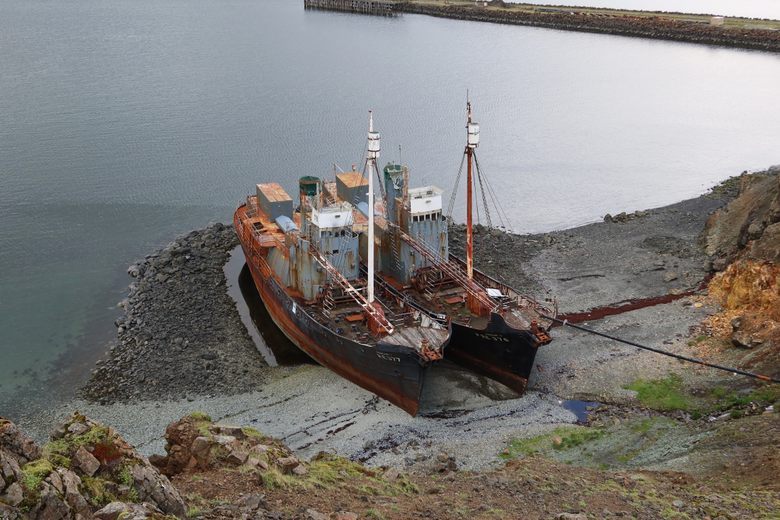On a dreary, cloudy day, this photograph captures a serene, almost eerie coastal scene from an elevated perspective. The calm, glassy water stretches into the background, highlighting the overall grayness of the day. In the foreground, two ancient, rusted fishing boats are beached side by side on a rocky, sandy bank that juts out like a manmade projection, covered in a mix of gray rocks, clay, and sparse mossy greenery.

The boats, with their dark, almost black, rust-covered bottoms and reddish-orange, corroded fronts, stand as ghostly relics from a bygone era. One of the boats features two prominent poles, one white and less rusted, the other more corroded, with multiple cables hanging down. The backs of the boats are blocky and flat, resembling barges more than traditional ships, with split V-shaped tail ends and flat decks.

There are no signs of human activity around these derelict vessels, which appear anchored in or stuck on the mound of crushed stone, creating a hauntingly still and silent image of abandonment and decay.